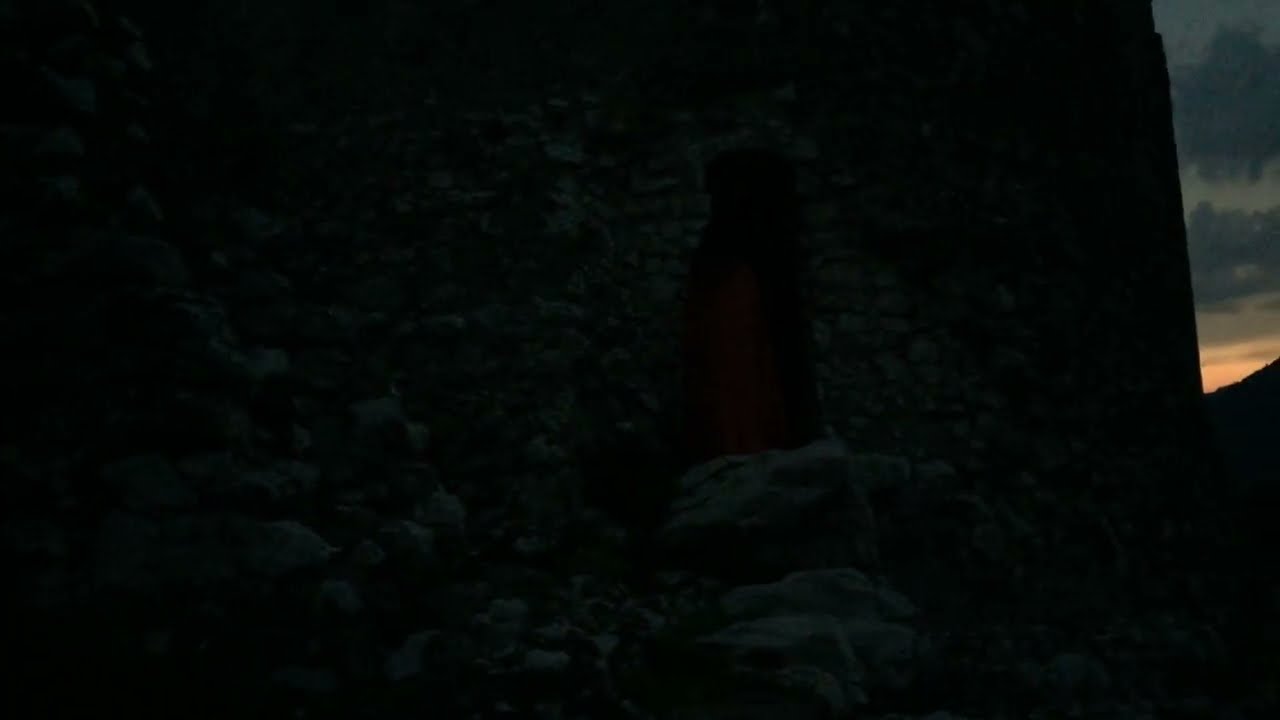This photograph captures a predominantly dark scene, with a close-up view of a large, irregularly shaped stone formation that seems almost dome-like but without the top visible. The stone surface is rugged and uneven, covered with numerous cracks where sparse greenery grows, contributing to the natural, gritty aesthetic. On the bottom right, within the stone structure, there appears to be an intricate arrangement of rocks, one balanced atop the other, and perched on this arrangement is what seems to be the silhouette of a black bird, possibly with a bright red breast, looking skyward.

The backdrop of the image, visible predominantly in the upper right corner, showcases a dusky sky with a mixture of dark grey clouds and a subtle hint of orange, indicating either an early sunrise or a setting sun. The light from the sky adds a faint illumination to the scene, casting shadows and highlighting the textures of the stones. There is also the silhouette of another hill or ridge far off to the right, adding depth to the overall landscape composition. The combined hues of gray, green, black, and red dominate the scene, creating a moody, almost somber atmosphere in what appears to be a desert-like environment.